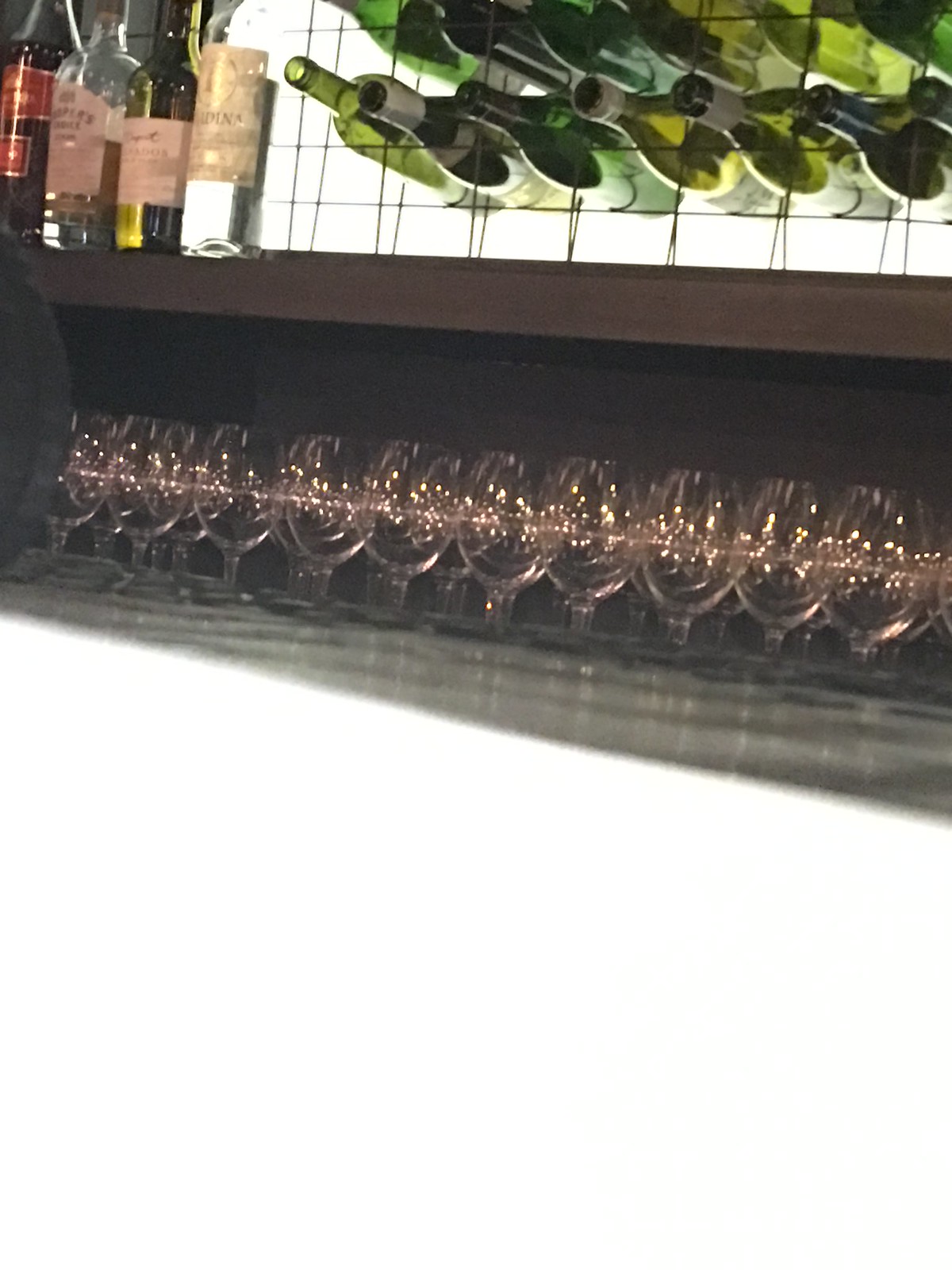This indoor photo captures a detailed view of a bar area with a grey countertop lined with numerous small wine glasses, each distinguished by their short stems and highly polished, shiny surfaces. Above the countertop, a wine rack made of a wire grid creates a tic-tac-toe pattern with square compartments that hold various wine bottles horizontally. The wine bottles in the grid exhibit an array of green shades, including dark green, light green, olive green, and bluish-green. On the top ledge of the counter, an assortment of liquor bottles stands, featuring clear bottles with red labels, one with a white label in a green jar, another with a white label in a clear jar with clear liquid, and a bottle with brown liquid adorned with a shield-like white label. Reflective lights shimmer off the glasses and bottles, adding a lively, illuminated ambiance to the scene.